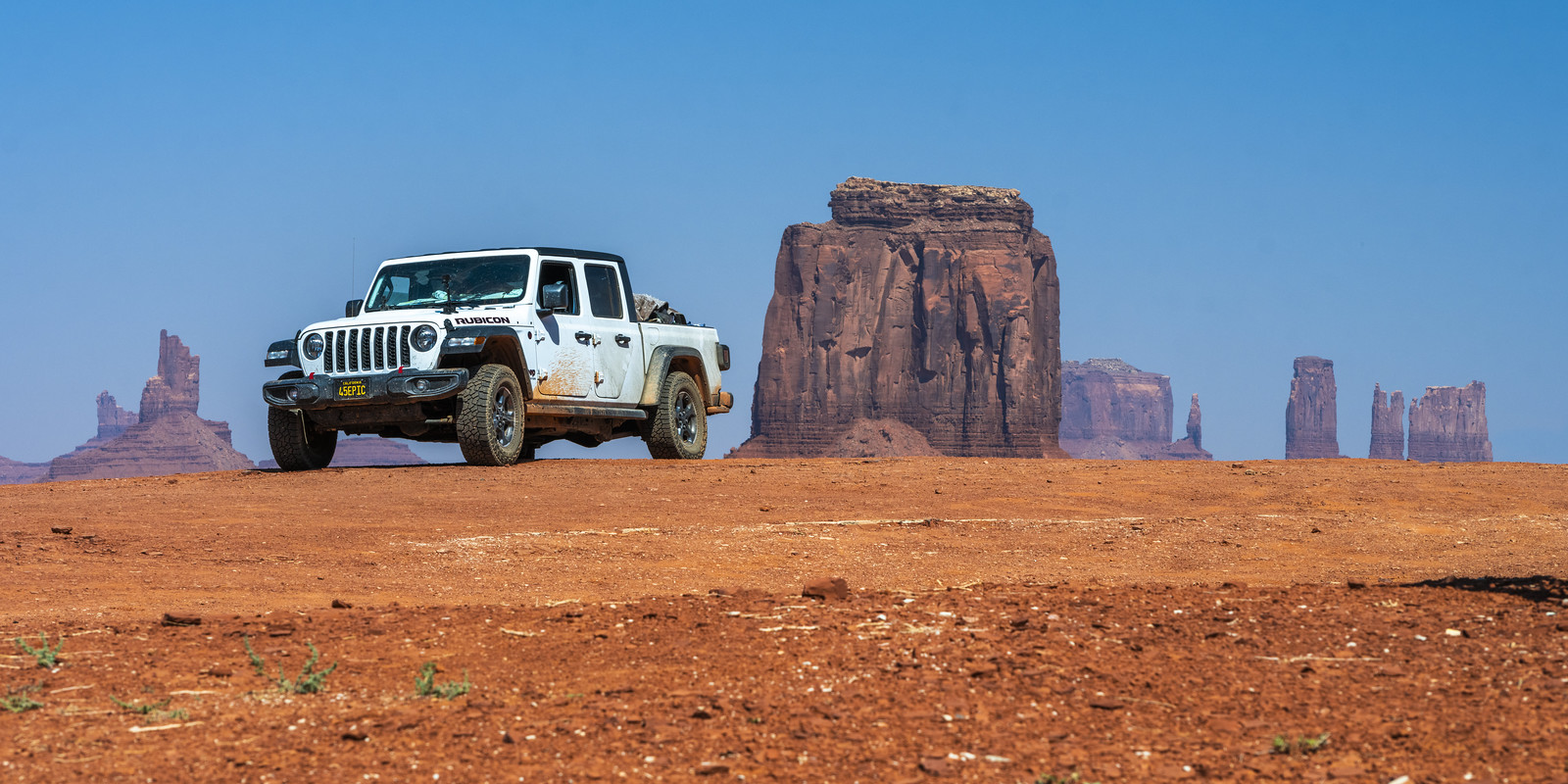The outdoor scene captures a stark and beautiful desert landscape bathed in the brilliant blue of a cloudless sky. In the middle left of the image stands a striking white Jeep Rubicon, distinguished by its black fender flares, black bumper, and unique truck bed design, revealing a load of rocks. The ground beneath it is a rugged expanse of reddish-orange sandy soil, speckled with red stones, contributing to the arid desert vibe.

The background features an impressive array of stone ridges and rock formations, stretching across the horizon. The formations are notable for their variation in height and width, with the tallest to the right of the Jeep and progressively shorter and wider structures flanking it. These rock figures exhibit a variety of jagged and smooth tops, giving them a unique feather-like distinction. The stones themselves are characterized by horizontal strata, adding to their textural and visual interest.

Sparse green plants dot the foreground, contrasting the otherwise barren, red-dominated terrain. The rugged scenery and the distinctive stone formations suggest that this photograph might have been taken in a region similar to Arizona or New Mexico, known for their majestic desert landscapes.